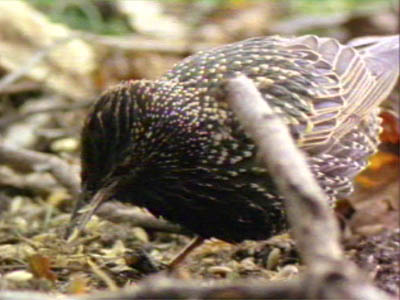In this detailed photograph taken outdoors on a cloudy day, a very small bird is prominently featured in the front and center, standing amidst ground debris that includes leaves, twigs, nuts, and mulch. The backdrop is slightly blurred, with green leaves at the top and a variety of colors like tan, yellow, orange, and white scattered around, contributing to a natural and earthy setting. The bird, potentially a young one due to its small size and peculiar markings, displays a predominantly dark plumage with intricate details. It has a medium-length, sharp, pointed gray beak, and its cute, round head and folded wings are adorned with white and yellow spots, and feathers outlined in blue, purple, and a whitish gold hue. The bird's tail feathers reveal a deep lavender shade. It stands on slender legs with relatively large feet, and near its left, it appears to be pecking at some yellow and orange matter on the ground, possibly searching for food like breakfast. A Y-shaped stick, part gray and brown, can be seen under the bird, adding to the rustic charm of the scene.